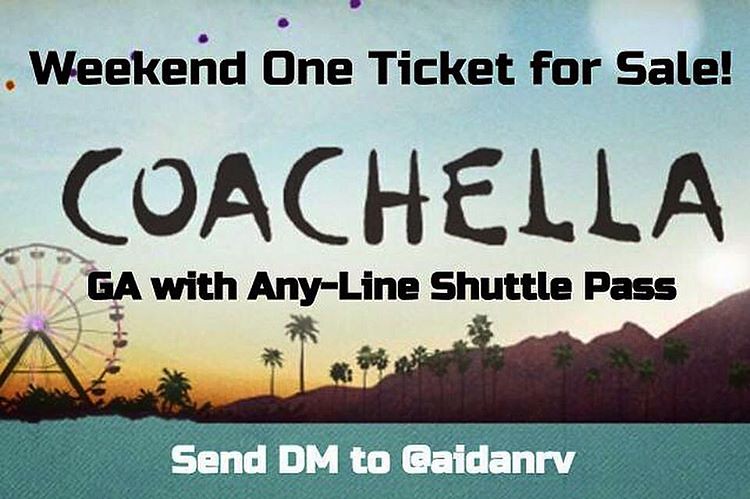The promotional flyer for the music event features a heavily edited photograph with vivid details. The backdrop showcases a majestic mountain peak in the distance, partially obscured by a light orange sky indicating dusk, with the sun peeking out from behind the mountain on the right. The scene is adorned with multiple palm trees in the foreground and a stylized cartoon Ferris wheel on the left. 

Overlaying this picturesque setting, bold black text spans the image, reading, "Weekend One Ticket for Sale, Coachella, GA with Any Line Shuttle Pass." At the bottom of the image, a blue border stretches from left to right, containing white text that instructs viewers to "send DM to @AidenRV." The flyer is punctuated with various hues, including shades of brown, green, pink, light blue, black, and white, creating a visually striking and detailed advertisement for the Coachella music festival.